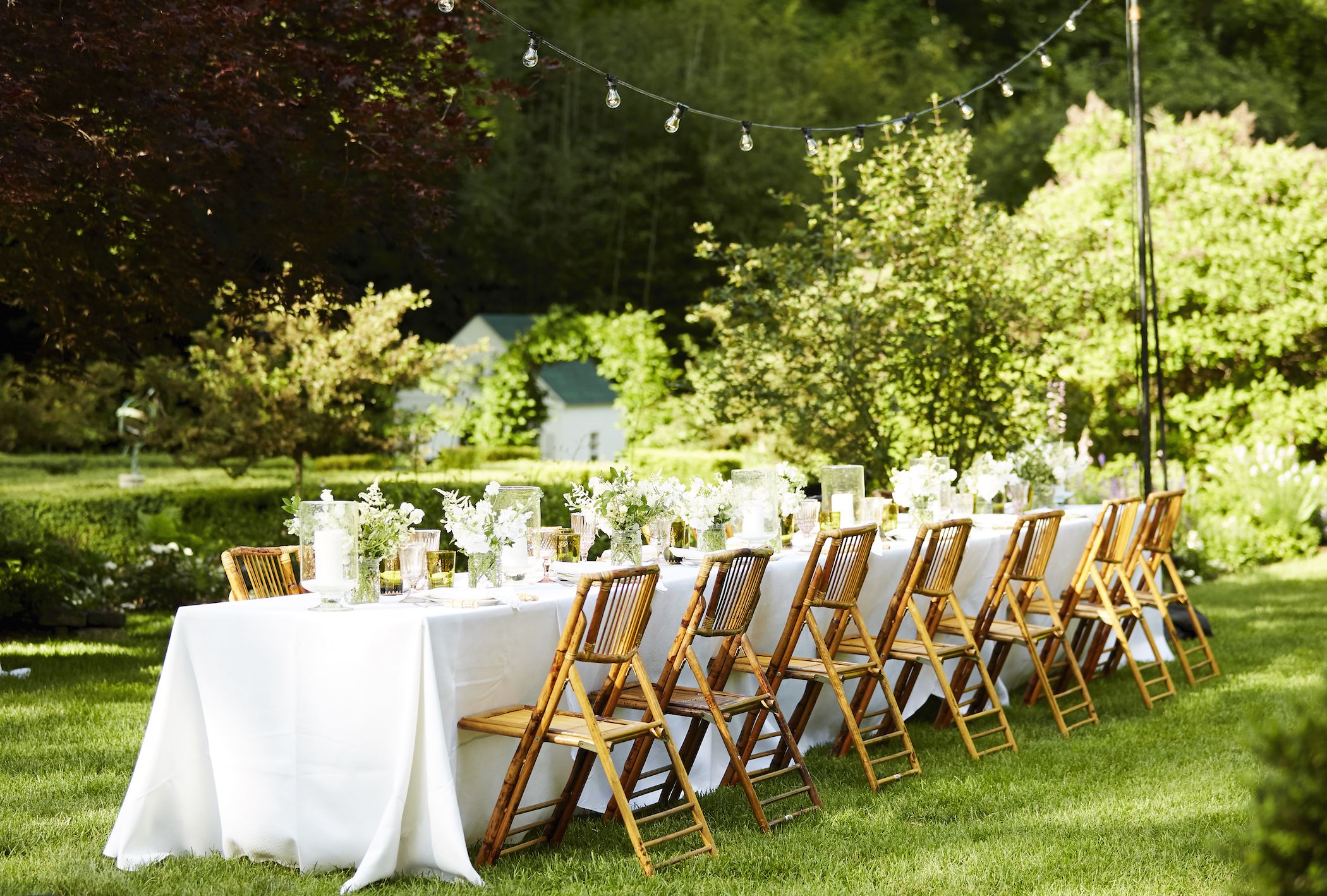The photograph captures a beautifully detailed, posh outdoor setting that appears to be arranged for a wedding picnic. At the forefront is an exceptionally long table draped in a pristine white tablecloth, set on a well-manicured lawn basking in sunlight. This table is flanked by fourteen light brown wooden folding chairs—seven on each side. The table itself is decorated generously with various vases, arrangements of greenery and white flowers, glass cylinders with white candles, and lace, creating an elegant and festive atmosphere.

To the right of the table, a mix of green and light white-colored shrubs and trees can be seen, their leaves glowing softly under the bright sun. Tall and distant, dense green trees form the backdrop, adding depth to the scene. On the left, a charming country house with white walls and a green roof peeks through, accompanied by a mix of greenery and a tree with brownish leaves. Above the scene, strings of Edison lights hang from an upright black pole at one end of the table, ensuring the area remains illuminated as dusk sets in. The overall ambiance suggests a meticulously cared-for space, perfect for a sophisticated outdoor celebration.